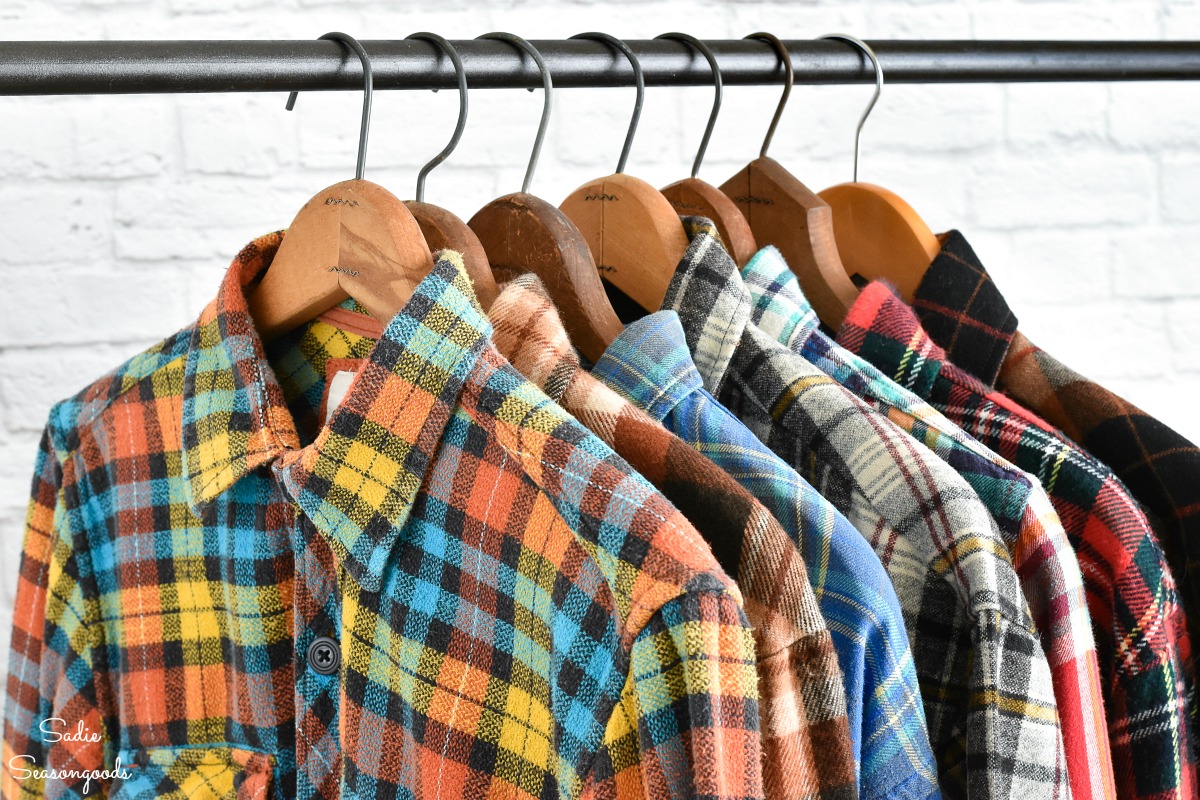The image features a close-up of a hanging rod set against a white brick wall background. Spanning horizontally across the upper portion of the photo, the black metal rod supports seven wooden hangers, each with silver metal hooks. Draped on these hangers are seven distinct plaid flannel shirts, all long-sleeved, adding a rich tapestry of patterns and colors. From left to right, the shirts display a spectrum of colors: the first shirt showcases a blue, orange, and yellow plaid design; the second incorporates brown, white, and tan hues; the third blends blue, yellow, and turquoise; the fourth has a mix of gray, yellow, and black; the fifth shirt introduces blue with hints of orange and white; the sixth shirt is characterized by red and dark green with white accents; and the final shirt on the far right intertwines brown and rust tones. All hangers are aligned uniformly, drawing focus to the shirts as they hang closely together, presenting a visually cohesive and vibrant array of flannel patterns. The indoor setting emphasizes the detailed textures and colors of the shirts, making them the central elements of the composition.